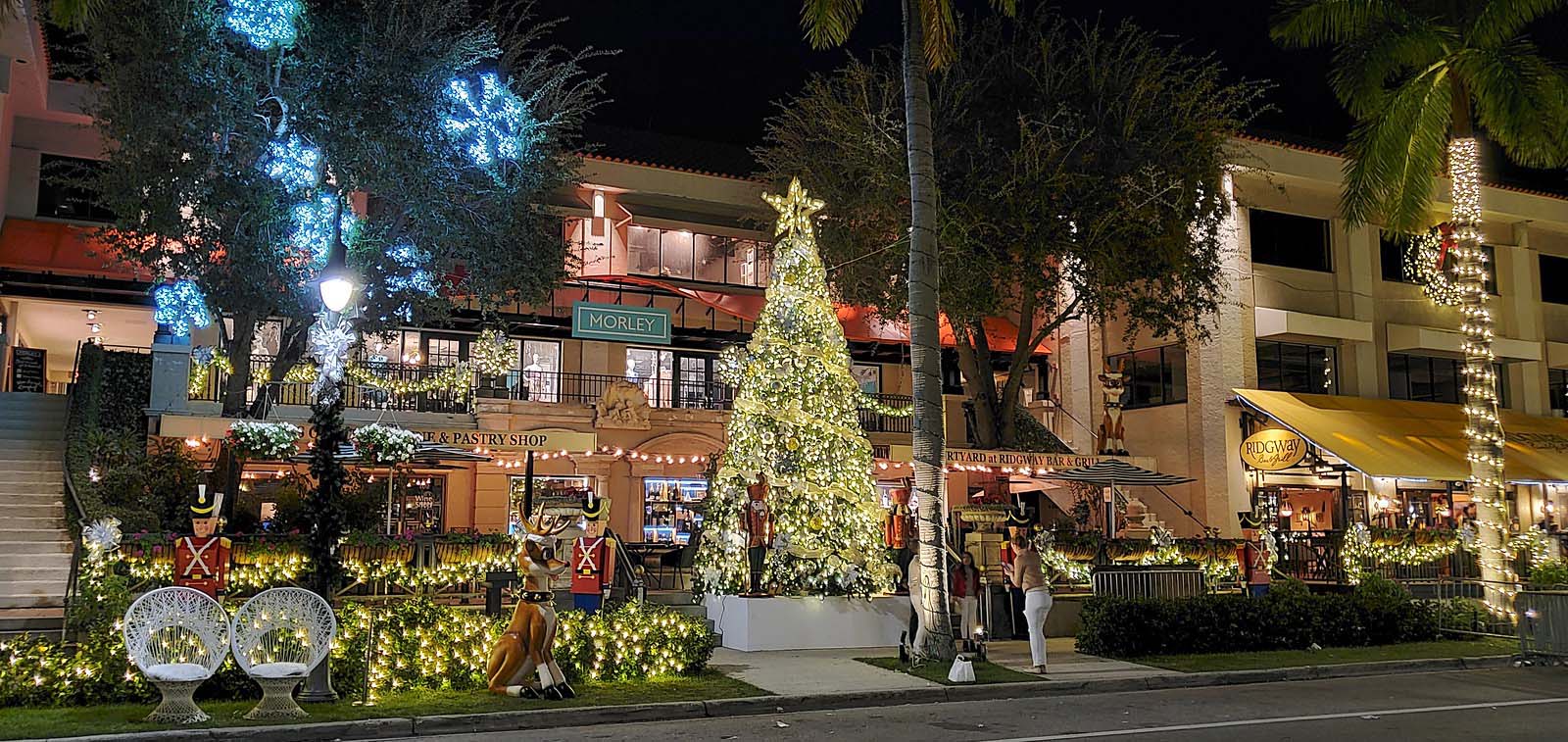This image captures a festive Christmas scene at an outdoor shopping mall, likely located in a warm southern locale such as California, Florida, or Hawaii. The scene is beautifully illuminated, highlighting intricate holiday decorations against the backdrop of nighttime. Central to the image is a towering, two-story Christmas tree adorned with white lights and crowned with a bright yellow star. Flanking the tree are life-size nutcracker statues and a reindeer figure posed as if seated like a dog.

The scene is bursting with holiday cheer, featuring a myriad of festive elements: bushes and railings decked with twinkling lights, palm trees with trunks wrapped in white spirals of illumination, and trees decorated with blue snowflake lights. A woman can be seen capturing a photo of two children, possibly with their father, in front of the dazzling Christmas tree.

To the left, two white chairs with lattice backs sit near a set of stairs leading up to a second-floor establishment, identified by a sandwich board suggesting a restaurant menu. On the right, a building displays a large lit wreath, while various shops can be seen in the background with signs reading "Mortley," "Ridgeway Bar and Grill," and "Pastry Shop." The overall ambiance is lively and warm, embodying the spirit of the holiday season with its sparkling decorations and inviting setup.